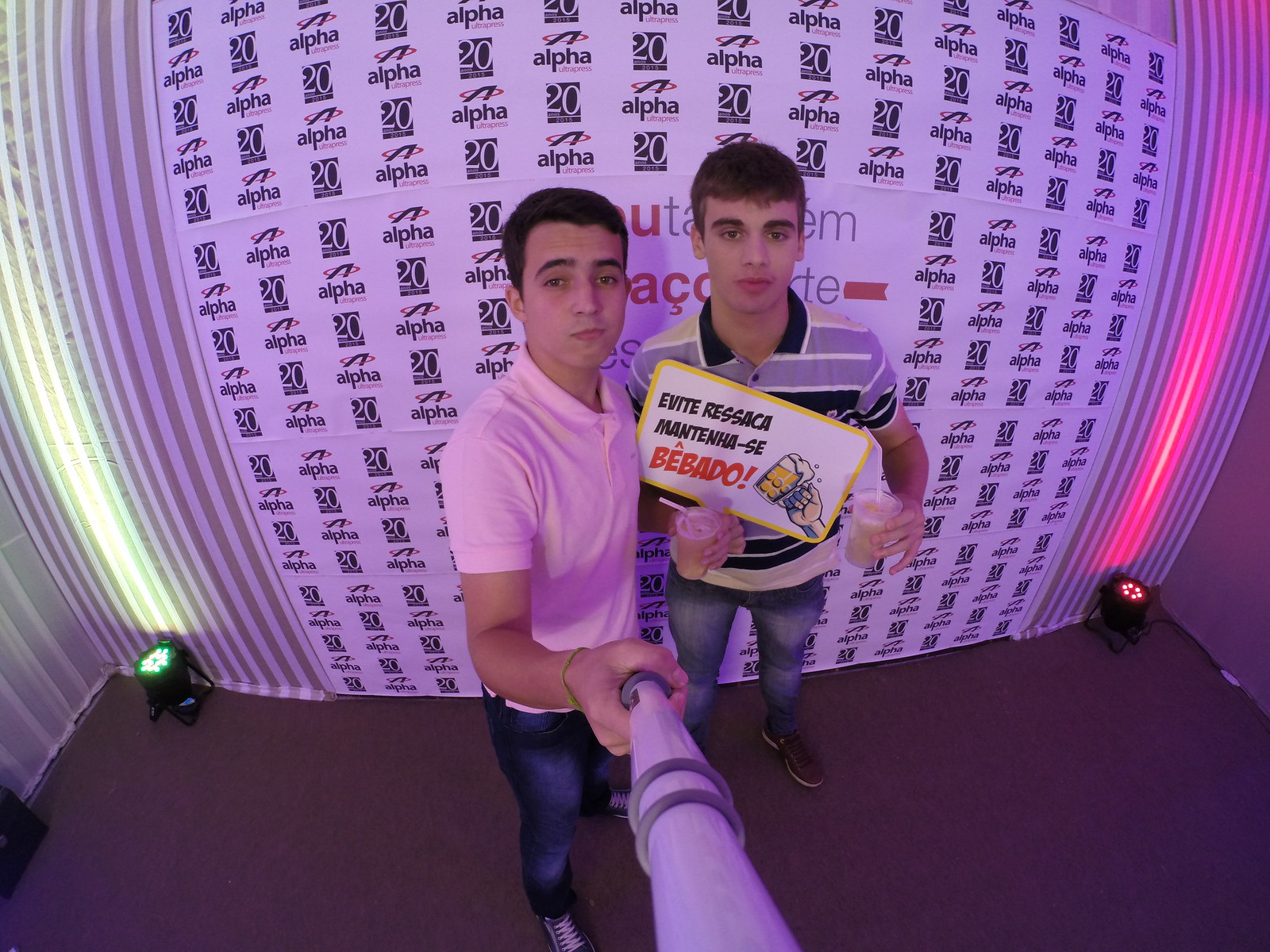This photograph captures two young Caucasian men standing close together, each holding a drink in a cup that looks like beer, though its light color suggests otherwise. They're dressed casually in polo shirts and tight blue jeans. The man on the left is wearing a pink polo shirt, blue skinny jeans, and Converse sneakers. He is holding a white selfie stick with two gray circles around the handle in his right hand. The man on the right sports a blue, white, and black striped polo shirt, and tight blue jeans. He holds a small yellow-bordered rectangular sign with Portuguese phrases: "Evite Ressaca Mantenha-se Bêbado!" (Avoid hangover, stay drunk!), along with a graphic of a hand holding a beer, foam spilling from the top. They are positioned in front of a white sign featuring a repeating pattern of the number '20' in white font inside blue boxes along with the word "alpha" in lowercase blue letters. The scene is set indoors, with a green light on the left and a red light on the right adding extra color to the backdrop.